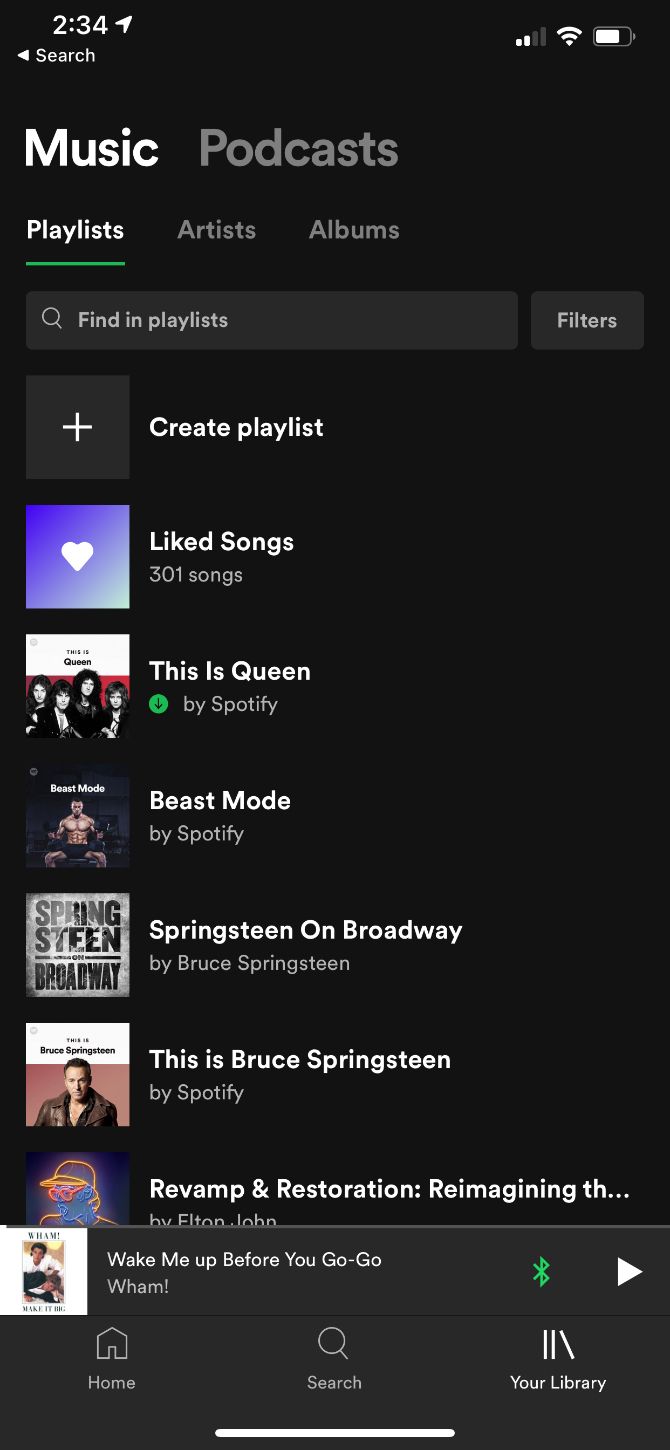The image depicts a Spotify interface on a mobile device. In the top left corner, the status bar shows the time as "2:34" with a signal indicator displaying 2 out of 4 bars, a WiFi symbol indicating a full connection, and a partial battery icon. Below the status bar, there's a search text field, and the screen reveals various music options under the Spotify app.

We see a "Playlists" section listing several categories:

1. **Queen by Spotify**: A dedicated playlist named after the band Queen, featuring the band members.
2. **Beast Mode**: A workout playlist indicated by an image of a muscular individual lifting weights. The playlist is curated by Spotify.
3. **Springsteen on Broadway by Bruce Springsteen**: A playlist showcasing Bruce Springsteen's performance, with an image of him standing.

Additionally, there's a gray search bar titled "Find a Playlist" with filters to refine the search results. A plus sign allows the user to create a new playlist. Visible on the screen is the currently playing song, "Wake Me Up Before You Go" by Wham!, next to a Bluetooth symbol suggesting the device is connected to an external audio source.